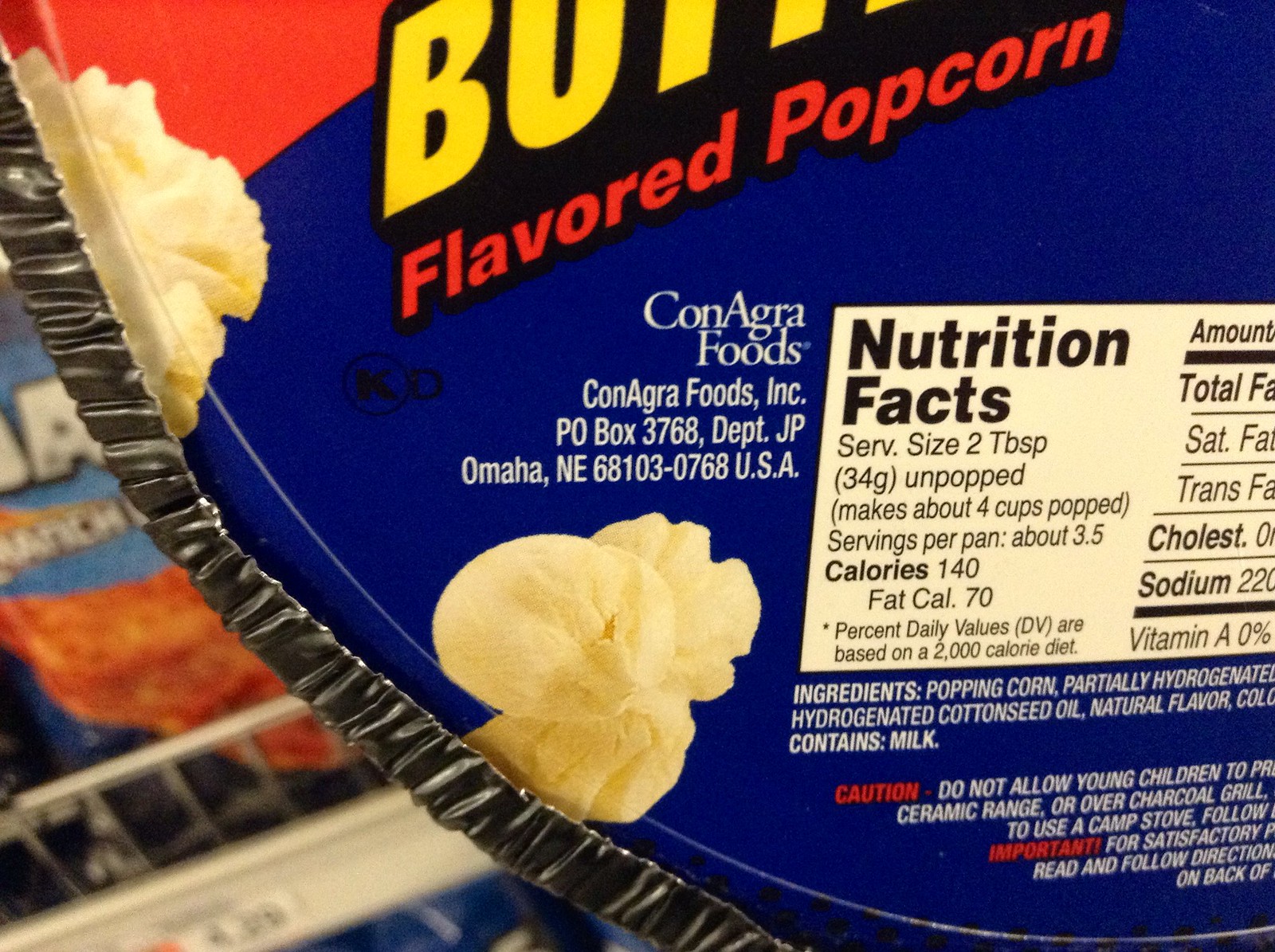This image showcases a pie-shaped package of butter-flavored popcorn, partially wrapped in foil with a thin cardboard cover. It prominently displays the brand "ConAgra Foods" and includes detailed nutritional information: serving size of 2 tablespoons (34 grams unpopped), yielding about 4 cups of popped popcorn, with 3.5 servings per package. The calorie count is 140, with 70 calories from fat. The ingredients listed are popping corn, partially hydrogenated oils, and natural flavor, with milk being a notable component. The package also features cautionary instructions regarding usage, specifically advising against allowing young children to handle the product. The photo, taken in a grocery store, also captures the bottom left corner of more items on the shelf. The package has a distinct blue covering.